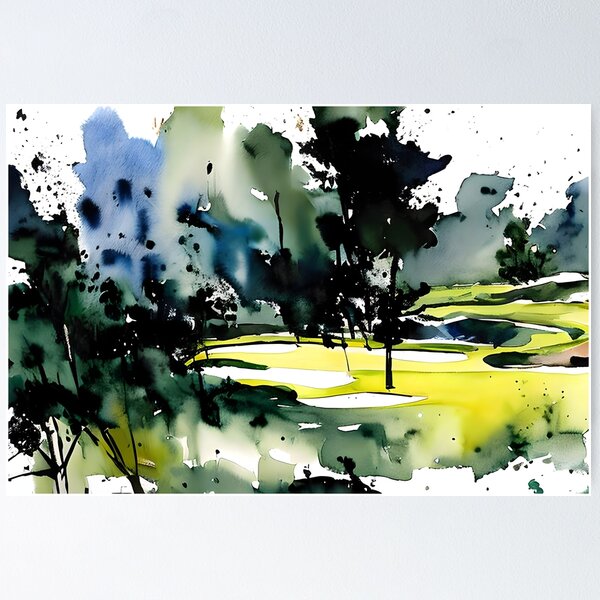The image is a rectangular watercolor painting with a predominantly white background, framed by gray borders on the top and bottom. Central to the composition is a scene that strongly resembles a golf course, featuring green fairways, sand traps, and possibly small ponds represented by white areas. The painting has an abstract quality, with elements appearing as though the artist angrily splattered black, blue, and green paint across the canvas. These splatters create a sense of chaotic energy, especially noticeable in the depiction of trees and foliage, which are rendered in black and appear almost dripping with paint. The left side of the image showcases more intense blue splatters, while the right side transitions to grays, with hints of yellow and beige scattered throughout. The background sky also shows a contrast between the left, which is more blue, and the right, which is grayer, with areas where the blue intrudes into the white, creating a smoky effect. Despite the randomness of the splatters, the overall impression is that of a golf course bathed in dynamic, abstract artistry.